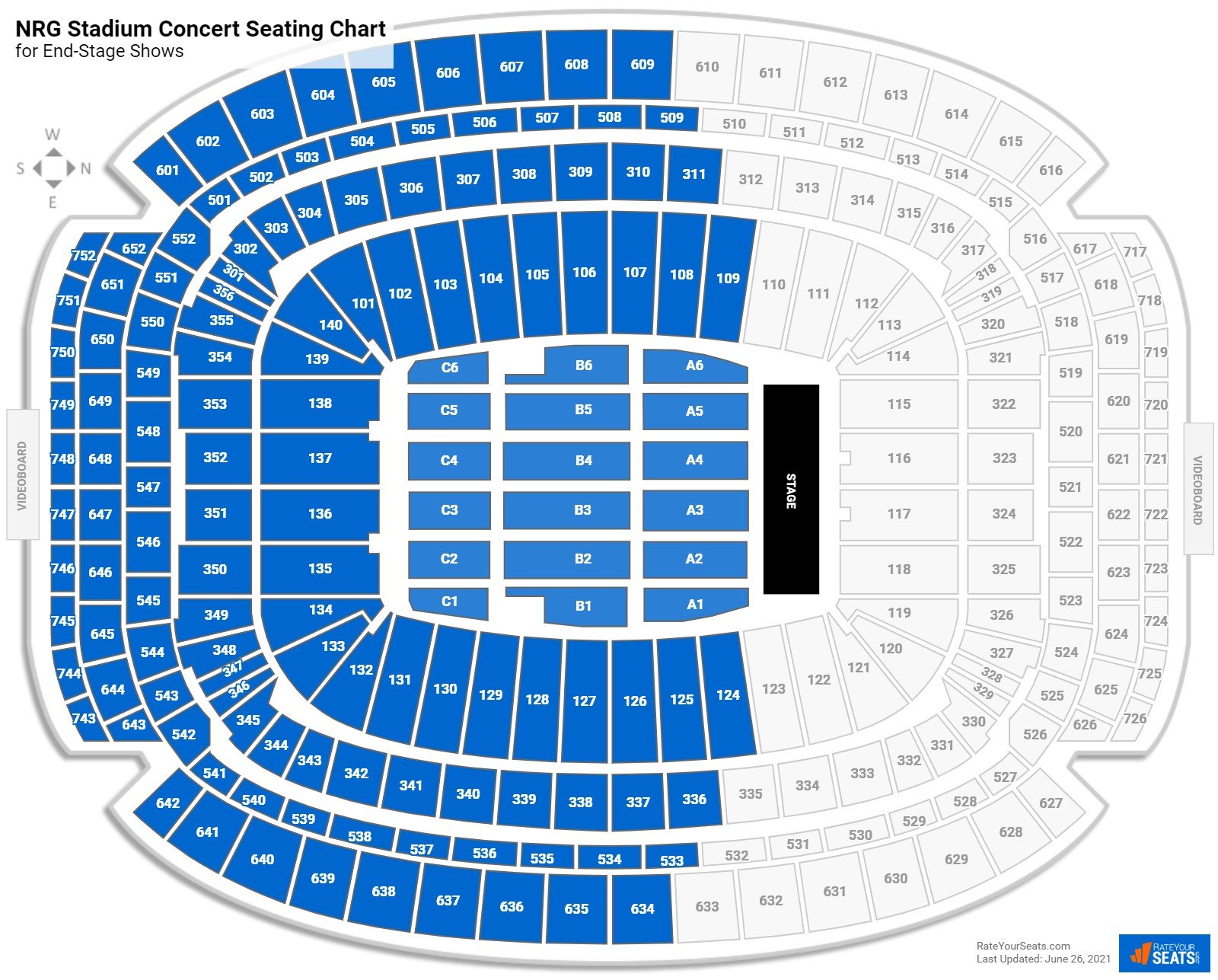This detailed digital image portrays the concert seating chart for NRG Stadium. Designed specifically for "N" stage shows, the diagram is a comprehensive guide for selecting seats during ticket purchases. The chart is color-coded, with seat sections filled in blue indicating available seats, and those in gray suggesting otherwise. Bold black text at the top labels it as the "NRG Stadium Concert Seating Chart."

A compass rose is displayed on the map to orient viewers, with a triangle pointing right for "N" (North), left for "S" (South), up for "W" (West), and down for "E" (East). The stadium layout showcases a black bar representing the stage situated towards the center. Seating sections encircle the stage, including some light gray seats positioned behind it, indicating they might have obstructed views.

Each section is meticulously labeled with alphanumeric codes for easy identification, such as A6, A5, A4, A3, A2, and A1, among others, encompassing the entire seating arrangement. At the bottom right corner of the image, a blue rectangle with white text stands out, featuring an orange logo. Adjacent to this, on the left, is a text box indicating the source "somethingyourseats.com", noting the last update was on June 26, 2021.